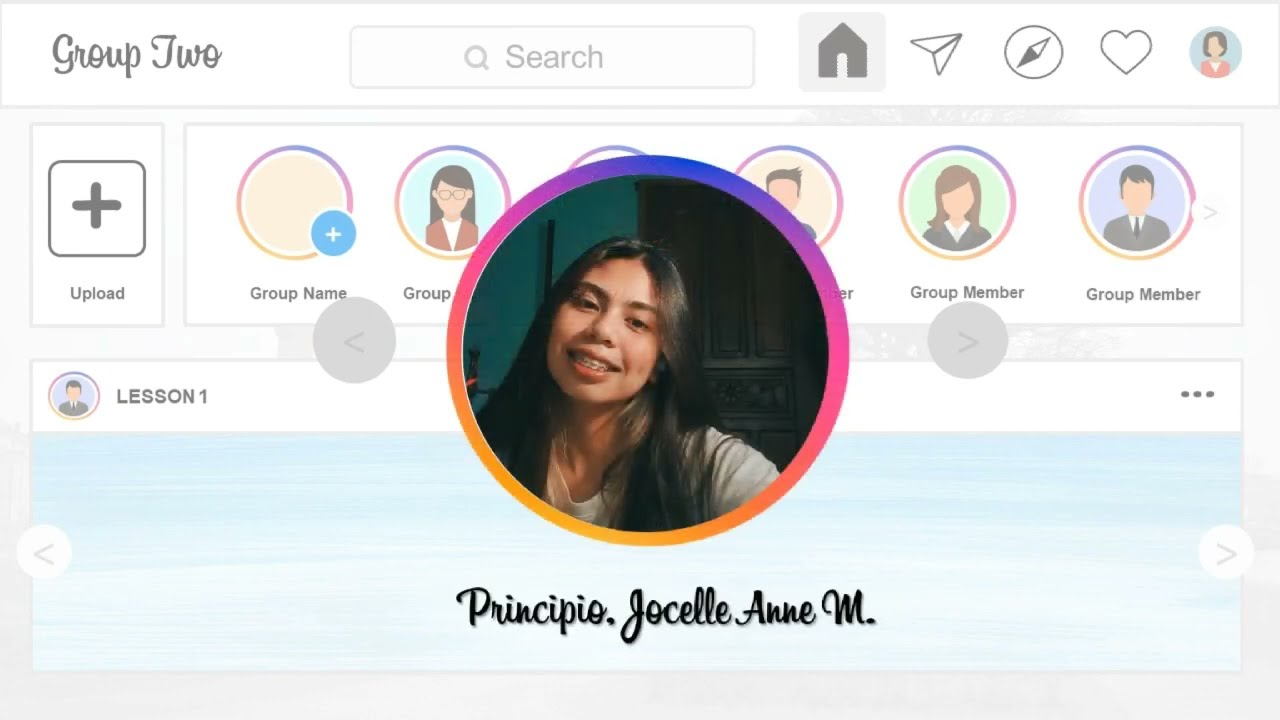The image depicts a screenshot of a social media app interface named "Group 2." The central focus is a circular photograph of a young woman with olive skin, wearing braces, and long black hair. She is smiling and wearing a grey top. The photo has a rainbow-colored gradient border, with hues transitioning through purples, blues, oranges, and yellows. The background of her selfie shows a dark wooden cabinet and turquoise walls. At the top left, there's the text "Group 2" in dark grey cursive, bordered by navigation icons including a home icon, a search bar, a share button, a locate button, a heart icon, and a profile thumbnail. Below the photo are additional icons like a plus/upload button and the text "Lesson 1" against a light blue rectangle. Below these is the text "principio.jocelynm" in cursive.